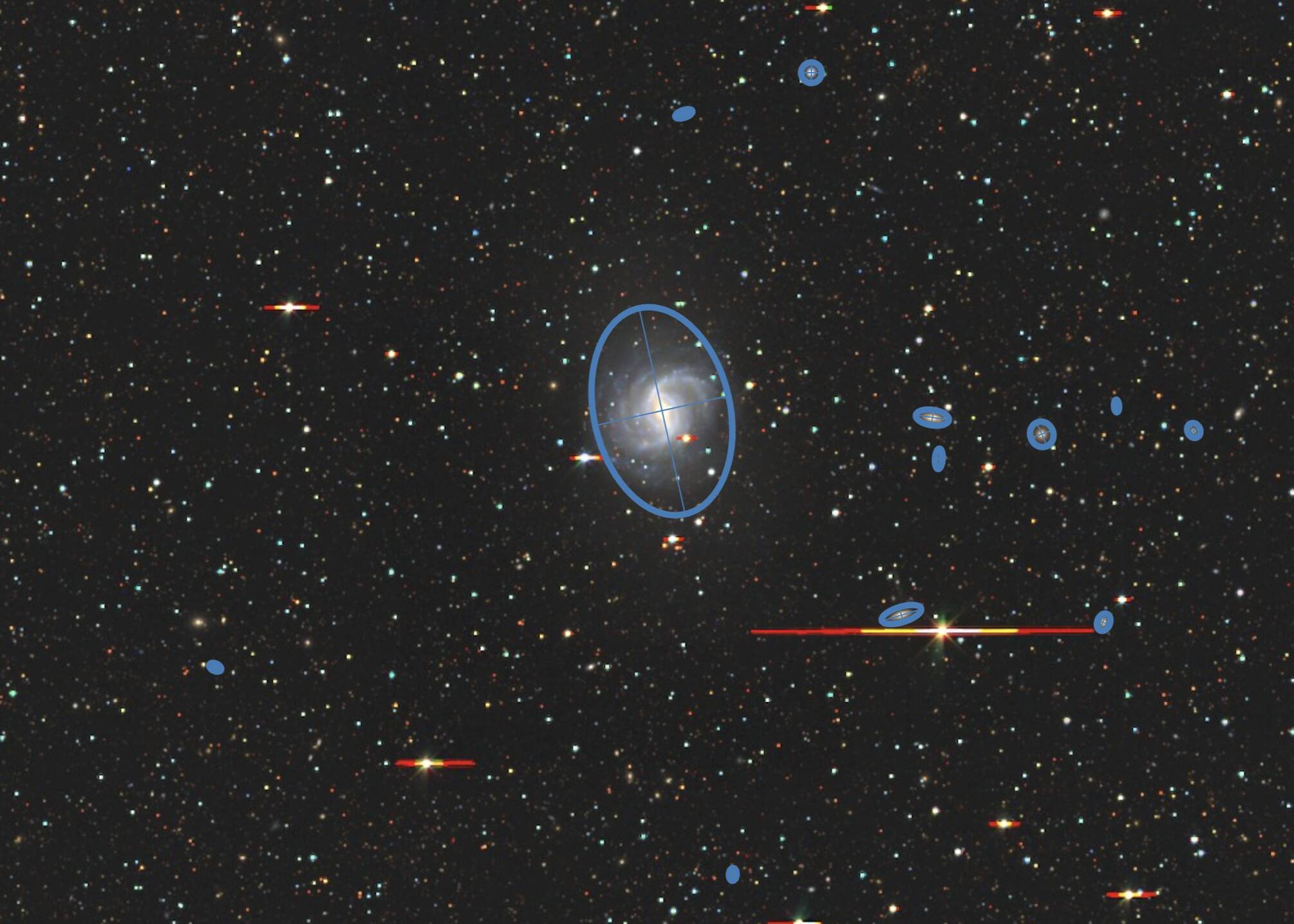The image depicts an expansive view of outer space, showcasing a vast array of stars scattered across the entire frame. Dominating the scene is a prominent galaxy, most likely the Milky Way, encircled with a distinctive blue target-like design complete with crosshairs. This central focus point is indicative of specific attention or analysis. Additionally, several individual stars and celestial objects are annotated with blue circles, highlighting possible planets or significant points of interest. The cosmos is interspersed with various colored markers, such as red and yellow, potentially denoting distances or other spatial data. The striking contrast between the luminous star clusters and the inky blackness of space further accentuates the depth and mystery of the universe. The entire composition conveys a sense of meticulous study or strategic mapping, akin to a scene from a sci-fi scenario or space exploration game.